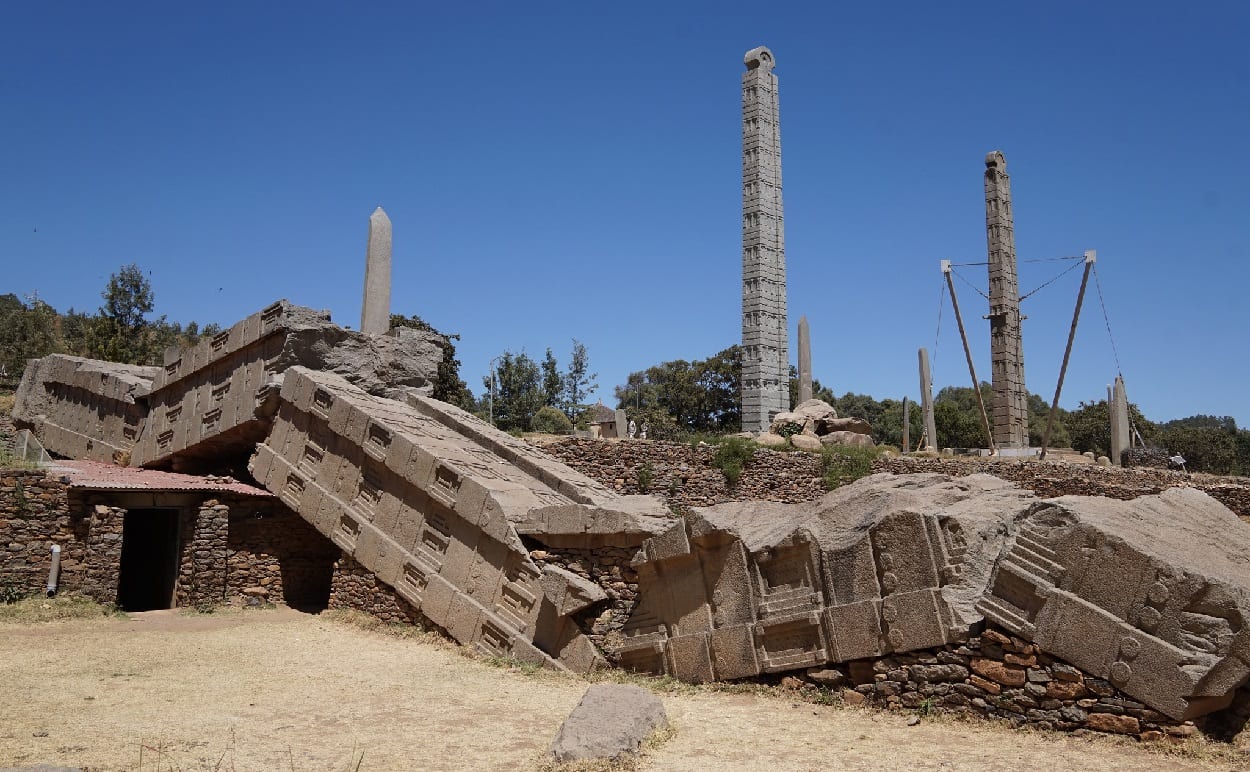The image depicts a collapsed structure in a desert landscape. In the foreground, brown dirt and sand lead up to a small hut on the left side, constructed of gray bricks. Above the hut, rubble from what appears to be a partially collapsed stone building cascades forward and to the right, breaking into four or five large pieces. Centrally, a decomposed structure resembling a bridge adds to the scene's chaotic atmosphere. Beyond this rubble stand three imposing gray pillars or obelisks, flanked by a few small green plants and tall gray towers. The backdrop is a line of trees stretching across the horizon, beneath a clear and cloudless blue sky. The image is devoid of people, animals, writing, and motorized vehicles.